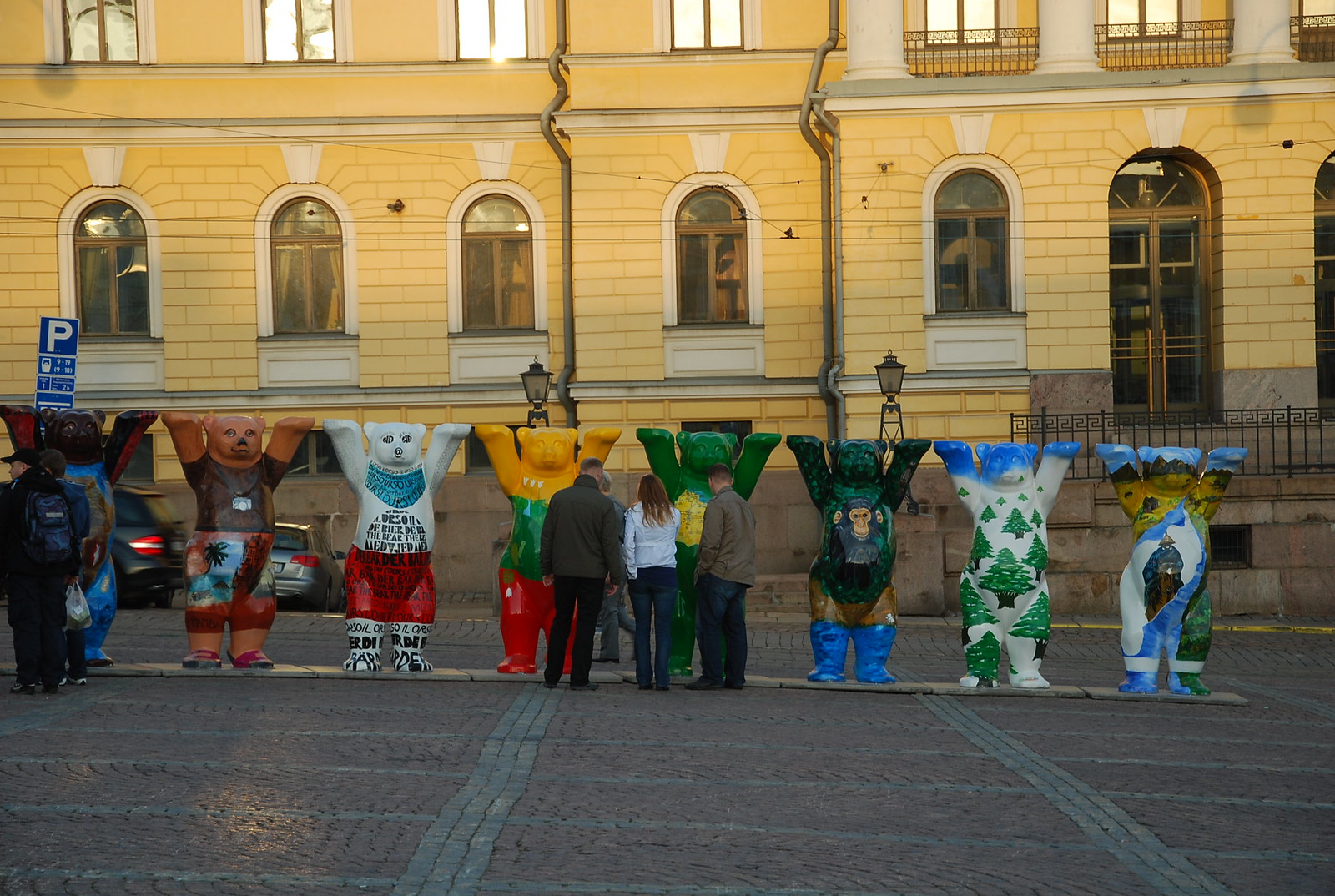This is an outdoor color photograph, likely taken at dusk or early dawn, showcasing a row of eight bear figurines standing on their hind legs with their paws extended skyward. Each bear is uniquely painted with a variety of colors and intricate designs. For instance, one bear is predominantly white with a blue head and paws, depicting a sky, and green pine trees arranged in a perspective that suggests a snowy landscape. Another bear features a gradient of yellow-orange on top, transitioning to green in the middle, and red at the bottom. Additionally, there is a bear adorned with red shorts, a blue bandana, and black text scrawled across its body. These figurines are located on a raised concrete strip amidst a cobblestone street, in front of a large, multi-story yellow brick building accentuated with arched windows and capstones. In the foreground, three adults—one woman in the center flanked by two men—stand with their backs to the camera, observing the bears. The scene is vibrant, with the street bustling with people examining the art.